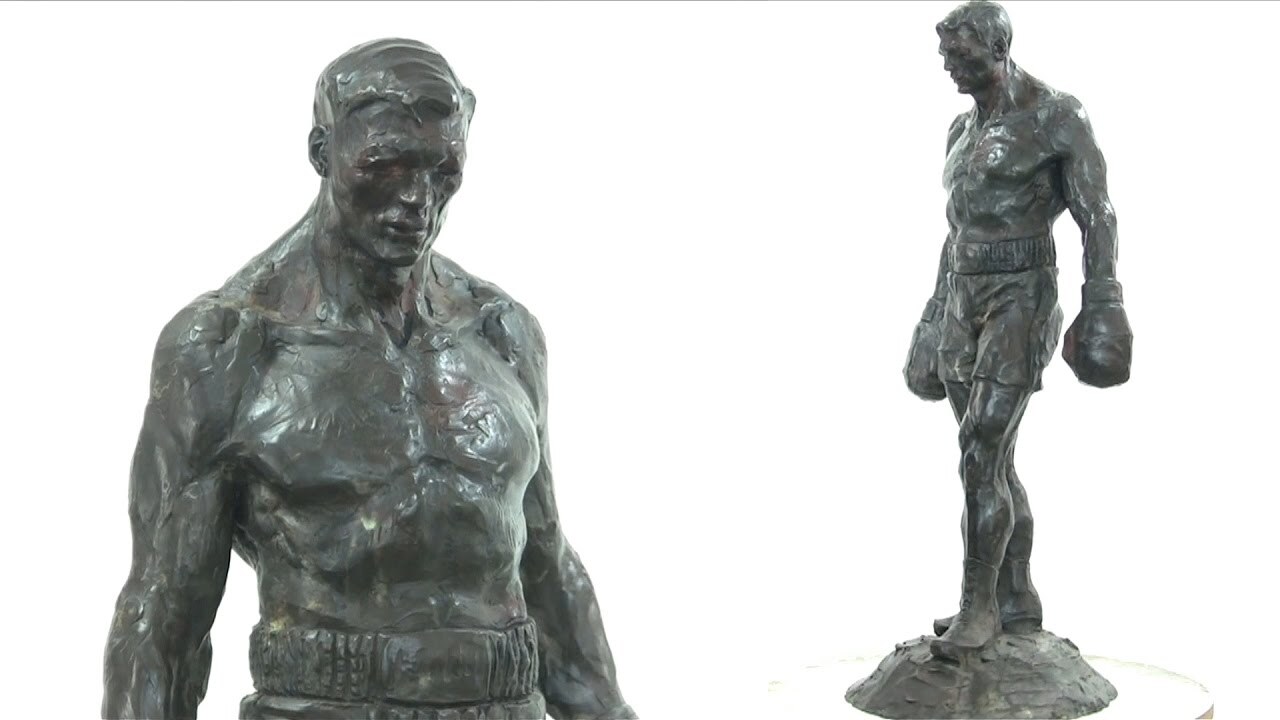The photograph presents two different angles of a bronze-like, dark green statue of a boxer, set against a white background. The first image captures a side view, featuring the boxer's combed-over, short-cropped hair, and muscular upper body, clothed in high-waisted boxing shorts reaching above the navel. The details of the face reveal a pensive, downcast gaze, possibly reflecting the aftermath of a lost fight. The second image offers a full-body view of the boxer standing on a small mound, showcasing his boxing gloves, shorts, and muscular legs in a dynamic stance with his left leg forward and arms poised in a fighting position. The handcrafted textures and lines give the sculpture a clay-molded appearance, embodying the essence and spirit of a determined fighter akin to the iconic Rocky Balboa.